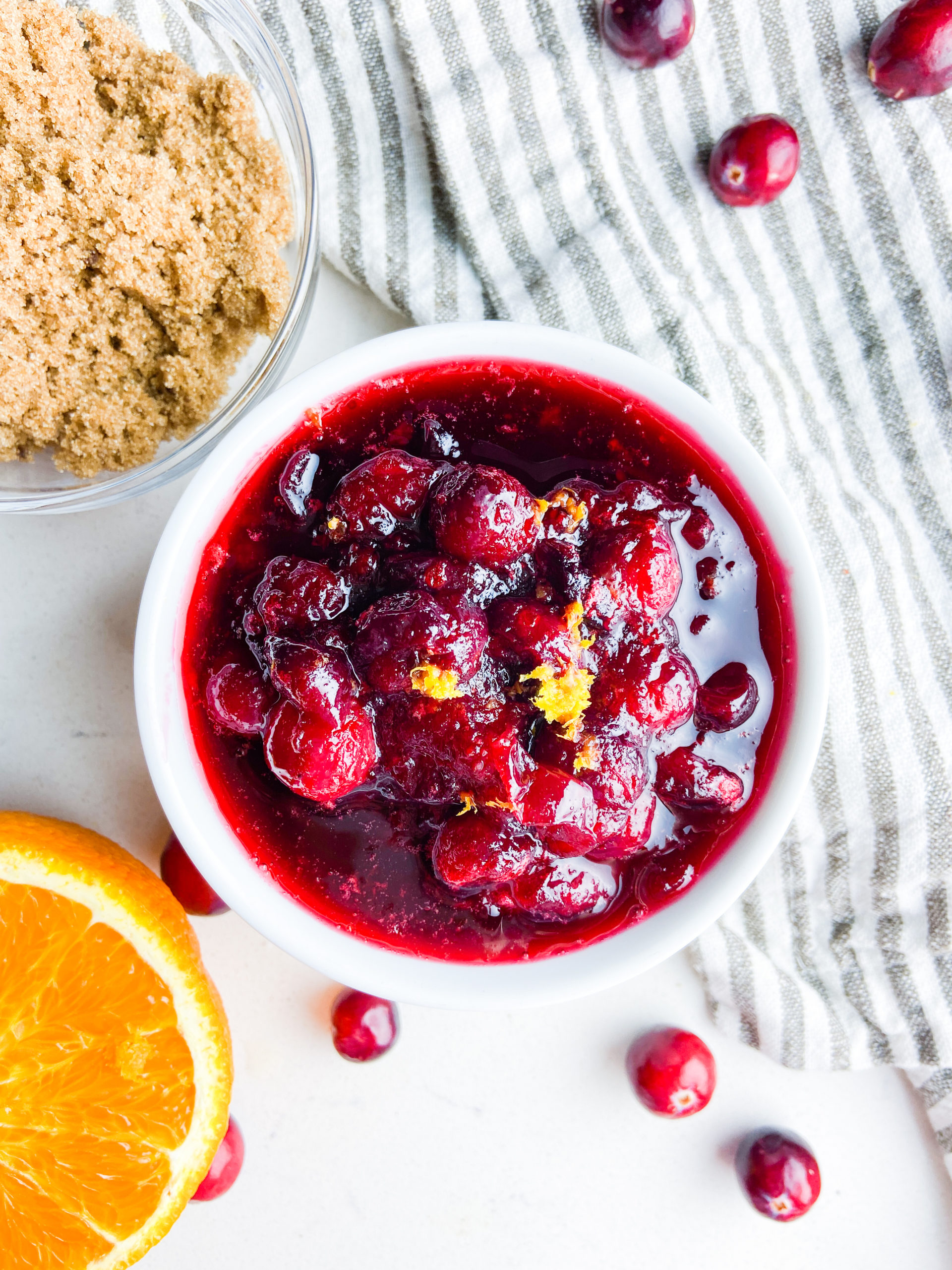Against a pristine white backdrop, this image presents a meticulously arranged tabletop scene dominated by a central white bowl brimming with vibrant red cherries immersed in a rich red juice. Nestled on a white surface, the composition is further embellished with loose cherries scattered around the table. To the left of the main bowl, a halved orange adds a splash of bright citrus color. Adjacent to this, there's a clear bowl filled with a tan cereal-like food, its ambiguous nature contrasting with the vivid fruits. A gray and white striped cloth, possibly a napkin, rests at the top right, adding texture to the overall aesthetic. The setting, devoid of any visible text, likely depicts an indoor environment, possibly a kitchen, with a color palette comprising predominantly of white, gray, red, maroon, brown, yellow, and tan. The meticulous arrangement and vivid colors create a visually appealing, almost serene scene suggestive of a quiet moment in a homely kitchen.